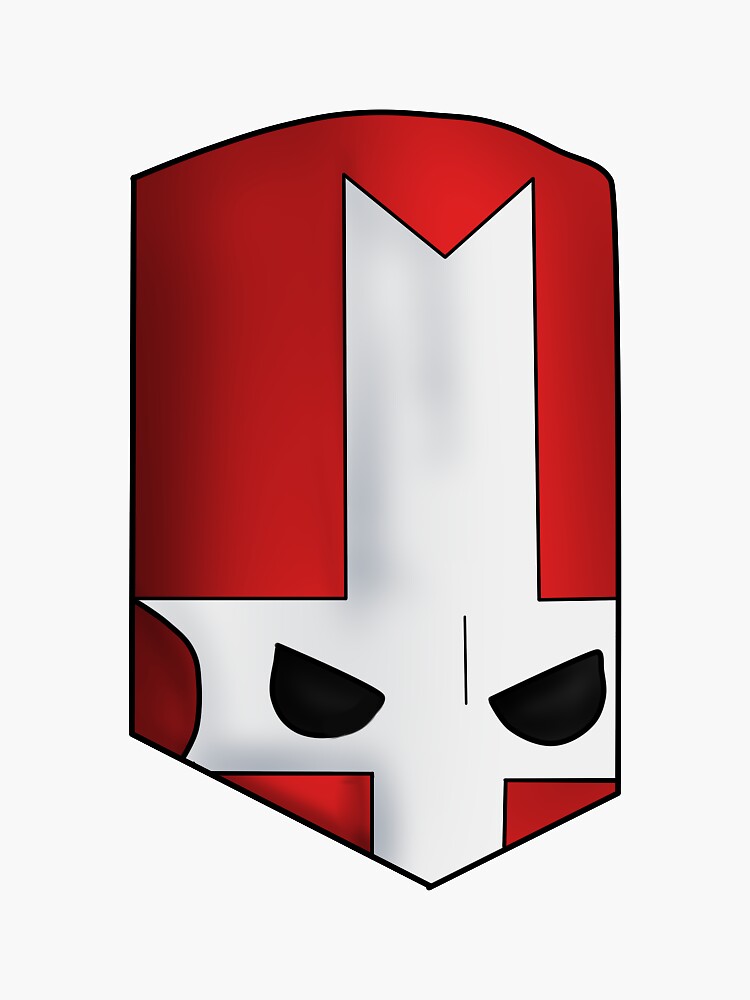This is a detailed caption for the image:

"A striking digital illustration shaped like an almost-shield captures the eye immediately. The illustration features a curved upper area, indicated by an arched top, followed by two straight lines that descend to slightly different endpoints. From the left point, a long line angles downward and then connects with a shorter line that inclines upward to join at the right endpoint, creating a unique, irregular border. This entire form, resembling an elongated cylinder, is filled with a deep red hue, accented with nearly black tones along the left side and transitioning into a vivid bright red in the center.

Within this peculiar and bold red shape, an inverted cross is prominently displayed. The apex of this cross features a V shape, with two straight white lines that extend downward. A horizontal crossbar intersects these lines, curving inward on the left side, adding an additional layer of complexity. Enhancing the menacing appearance, two half-moon shaped eyes are drawn within the structure, their outer edges tilted upward while the inner edges aim downward, providing a grumpy or angry expression that adds an intimidating and sinister feel to the entire illustration."